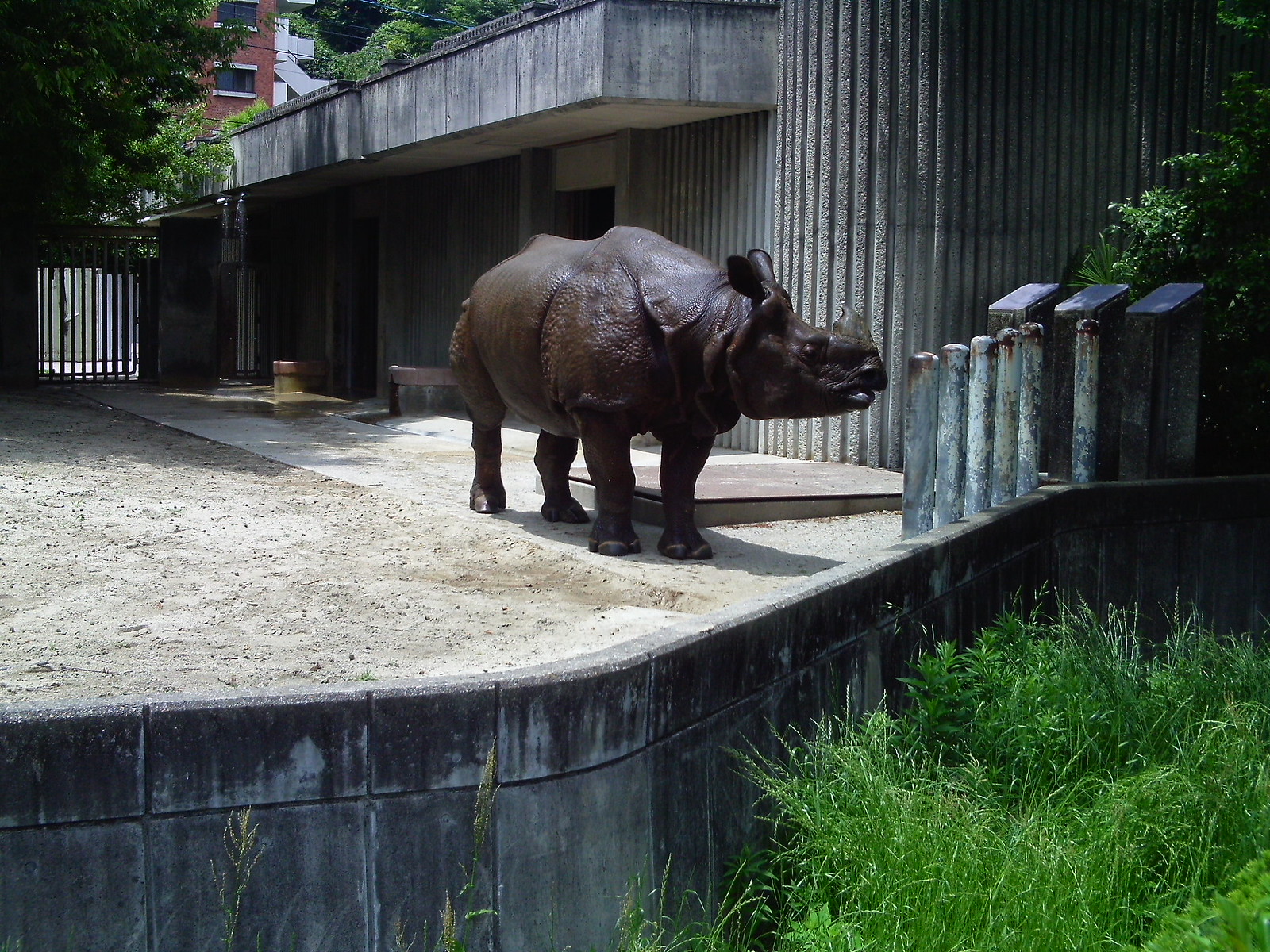This photograph captures a rhinoceros, possibly a statue due to its bronzy and shiny appearance, situated in what appears to be an outdoor zoo enclosure. In the foreground, long green grass contrasts with the grayish concrete wall of the animal's habitat. Metal pipes extend above this wall, suggesting structural support or barriers. The enclosure features a bare dirt and gravel ground, devoid of any greenery within. Behind the wall, there's a concrete building with an overhang, likely serving as a shelter for the rhinoceros. Trees and a much larger building are visible in the background. The rhinoceros itself is looking off to the side, displaying its partial horn, prominent ears, and segmented, armored-like body. The hoofed feet suggest realism, but the bronzy sheen leaves ambiguity regarding its authenticity.